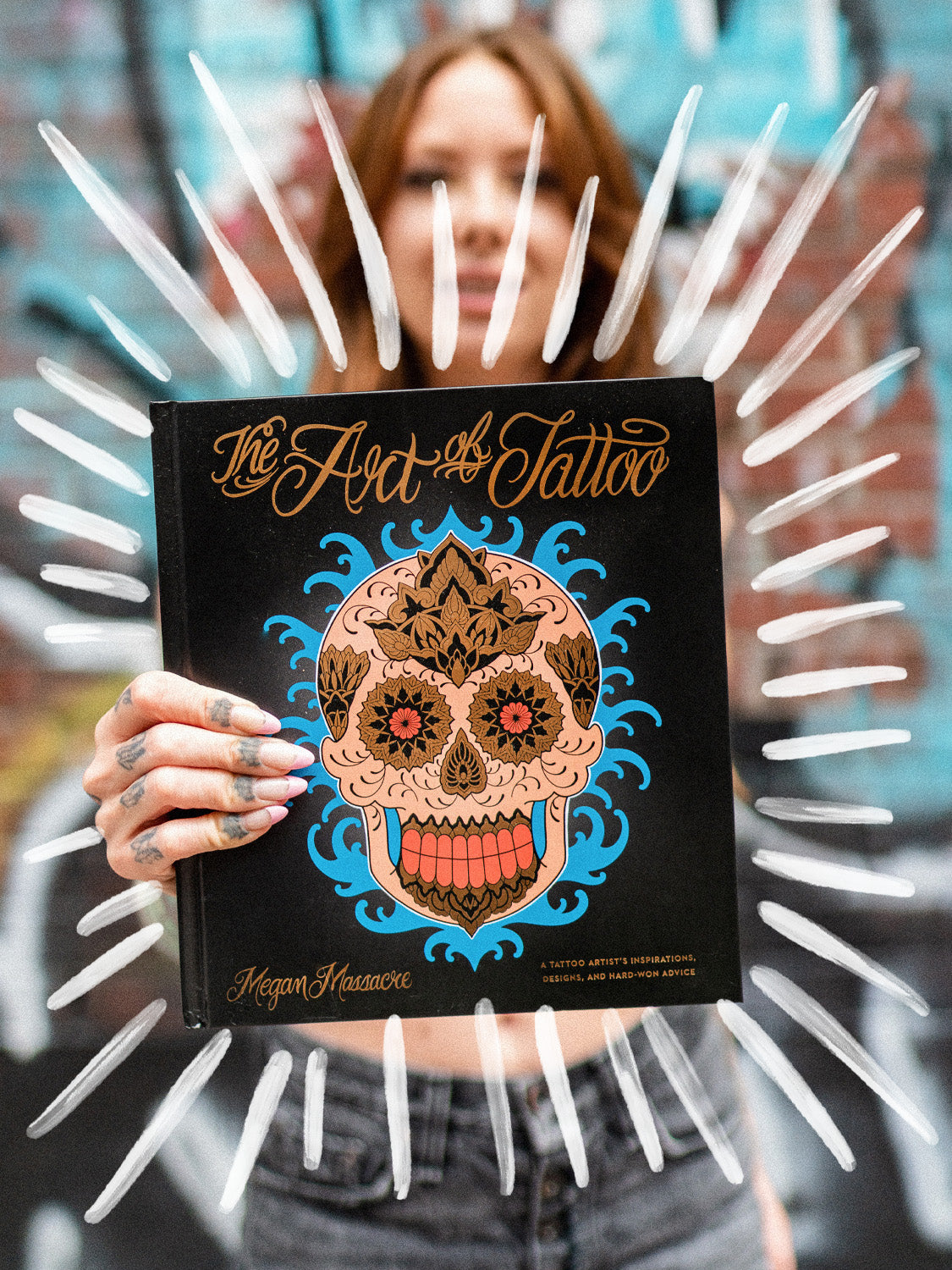The image depicts a young woman with light brown hair, standing and holding a book titled "The Art of Tattoo" by Megan Massacre. The cover of the book features a black background with an elaborate skull design that incorporates blue floral elements, giving it a glowing effect. The title, written in a golden handwritten style, appears at the top, while the author's name is positioned on the lower left side. The woman, who has tattoos on her fingers and is wearing dark-colored jeans, is blurred out in the background, making the book the focal point of the picture. The background is a blue hue, and white lines have been superimposed around the book to further emphasize it. The wall behind the woman is adorned with graffiti.